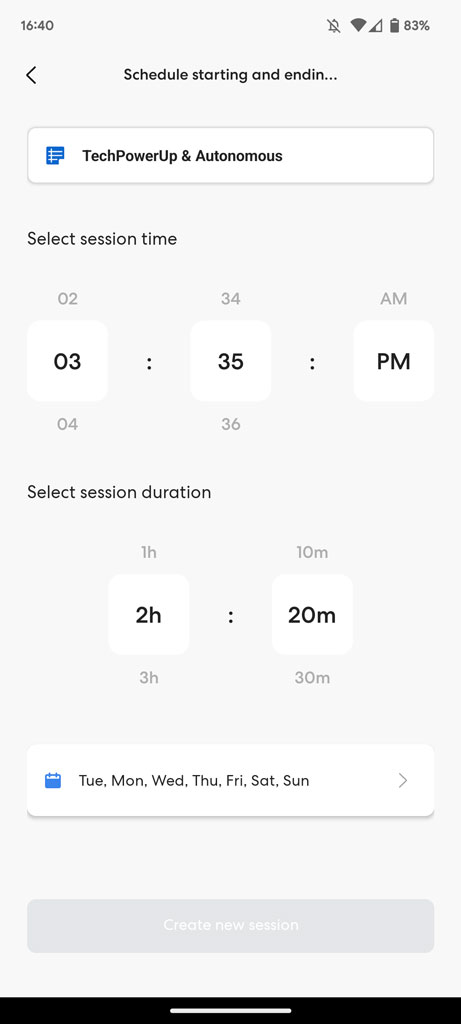This image, captured from a cell phone screen, features a predominantly gray background. At the top of the screen, there's a section labeled "Schedule Starting and Ending," followed by an ellipsis (…). Below this header, a search bar displays the query "Tech Power Up and Autonomous." 

Further down, there's an area labeled "Select Session Time" where the user has chosen a time designated as 03:35 PM, represented in three separate fields separated by colons. This selection indicates that the user has input "03," "35," and "PM" individually.

Continuing down, the image shows a "Select Session Duration" section where the user has set a duration of 2 hours and 20 minutes. This selection is displayed through a scrollable interface: "2H" is selected, with "1H" and "3H" serving as the options above and below, respectively. Similarly, for the minutes, "20" is chosen, flanked by "10" above and "30" below. This setup allows for easy adjustment of the session duration by scrolling.